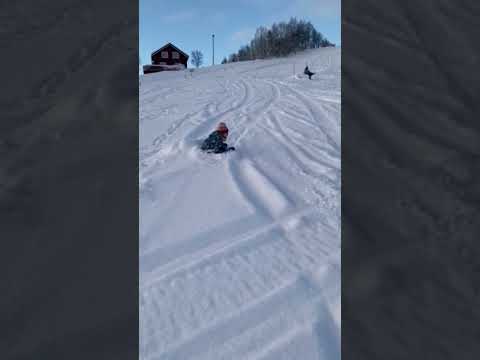The image depicts a snowy landscape segmented into three vertical sections. The left and right thirds are close-up views framed in black, focusing on different aspects of the snowy scene. The central section showcases a snow-covered slope with a prominent small brown house situated in the upper left corner, featuring two square windows above and snow on the awning below, creating a smiley face effect. Rising rightwards from the house are numerous leafless trees, while downward to the front are visible sledding tracks marking the hill. Slightly off-center to the left, a child is seen sledding down the slope, trailing a path in the snow. A crossing mark, possibly from a snowmobile, is noted at the lower end of the hill. The sky above transitions from blue to gray, adding to the wintery ambiance. Overall, the scenery is bustling with activity, as evidenced by the numerous tracks, suggesting many have enjoyed sliding down the hill.